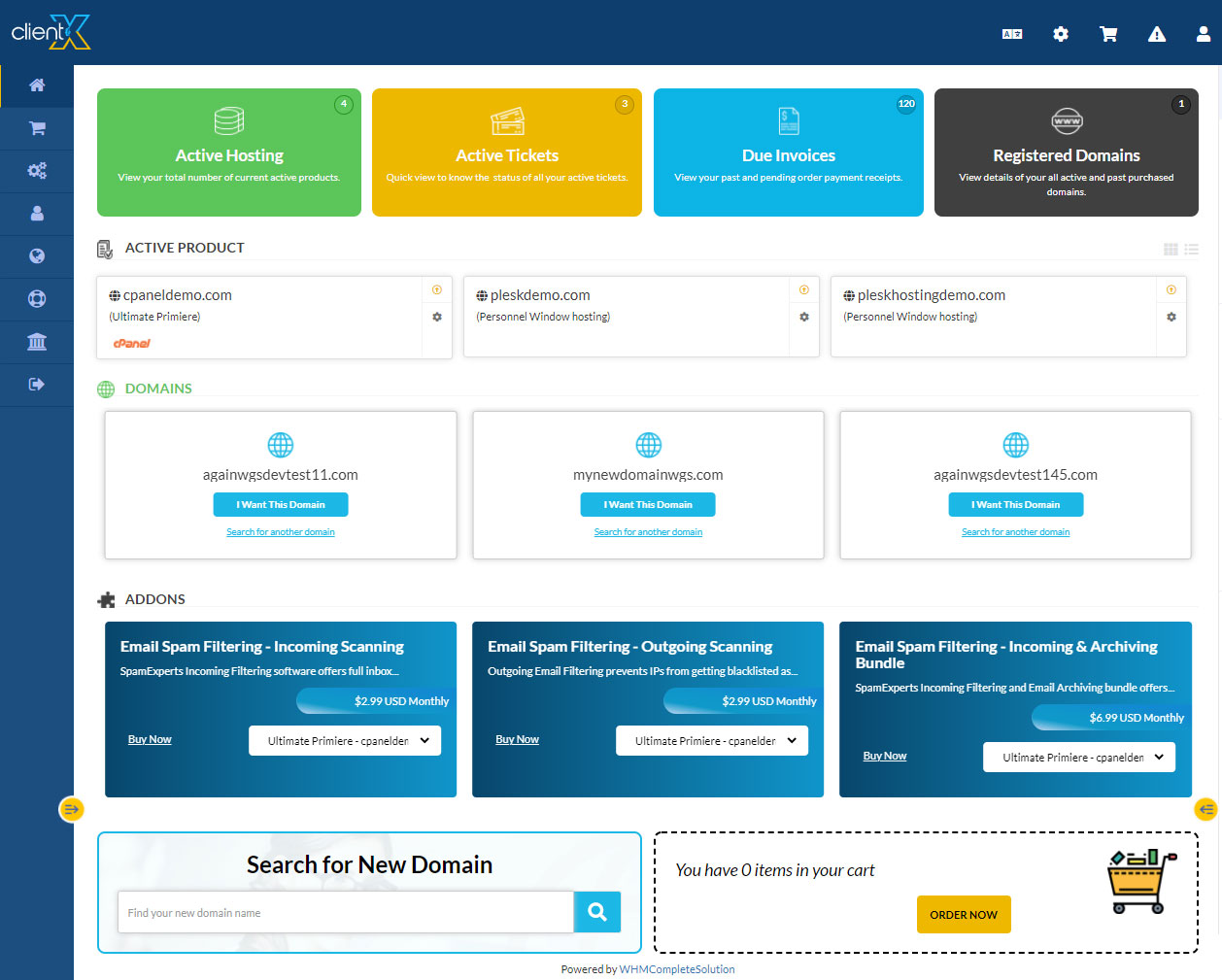This image showcases a detailed website interface for a client management portal named "Client X." The interface features a dark blue top navigation bar with the "Client X" logo on the left side. On the right side of this bar are icons for language settings, shopping cart, issues/settings, and user profile.

Along the left side of the interface, there is a vertical navigation bar in a slightly lighter blue color. This bar includes several icons underneath the "Client X" logo: a house icon (home), shopping cart icon (shopping), settings icon, profile icon, world icon (language settings), a lifeboat circle icon (support), a courthouse tower icon (legal), and a logout icon.

At the top of the main content area are four large, colored boxes serving as quick access categories:
1. A green box labeled "Active Hosting" with an icon of coins, explaining the total number of current active products.
2. A yellow box labeled "Active Tickets" featuring a ticket icon for quick status updates on all active support tickets.
3. A blue box labeled "Due Invoices" with a document icon, allowing users to view past and pending payment receipts.
4. A black box labeled "Registered Domains" with an icon of a globe and "www," detailing all active and past purchased domains.

Below these categories is a section labeled "Active Products." It includes three white boxes:
1. "cpaneldemo.com Ultimate Premiere" with the cPanel logo beneath it.
2. "plusdemo.com Personal Windows Hosting."
3. "plushostingdemo.com Personal Windows Hosting."

Next, there is a section labeled "Domains" in green, featuring a world icon. Below this, three blue boxes display available domains with an option to "I want this domain" and a prompt to search for another domain.

Following the domains section, there is an "Add-ons" label with three dark blue boxes offering services like "Email Spam Filtering," each with a "Buy Now" button and a drop-down menu for pricing.

At the bottom of the interface, there is a search feature labeled "Search for New Domain" on the left, which includes a search box and icon. On the right, there's a shopping cart summary stating "You have zero items in your cart" with an "Order Now" button and a shopping cart icon.